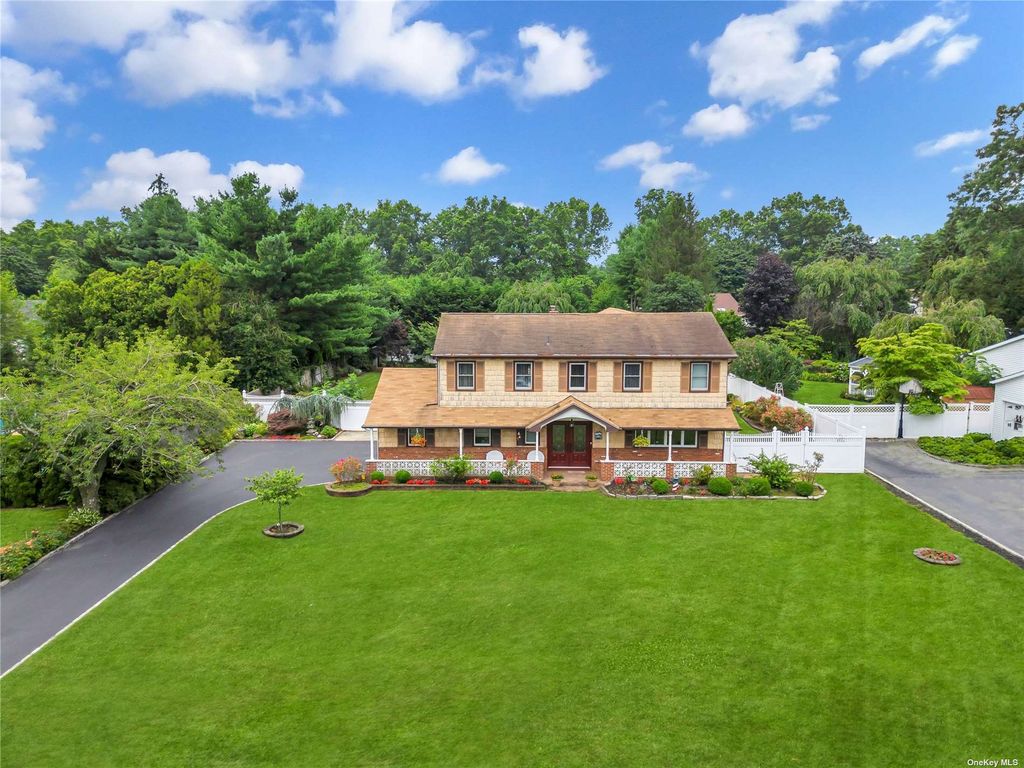This aerial photograph captures a large two-story house prominently centered amidst a lush, expansive lawn. The front yard is meticulously maintained, featuring a well-groomed green lawn that stretches broadly across the middle section, edged with tasteful landscaping. You can observe rings of stones marking the locations of small trees on both the left and right sides of the lawn, adding touches of nature to the otherwise open space. The house itself exhibits a blend of architectural details: its lower section is adorned with brick, while the upper story flaunts pristine white siding. A cozy porch, framed by a white picket fence, provides a welcoming entryway, complemented by twin maroon doors. Surrounding the house are low bushes, small trees, and beds of vibrant red flowers. 

The setting is encompassed by a backdrop of tall green trees, enhancing the tranquil suburban atmosphere. White picket fencing extends around the backyard, suggesting a harmonious blend of privacy and aesthetic appeal. The sky overhead is a brilliant blue, dotted with fluffy white clouds that add to the serene and picturesque quality of the scene. Driveways are visible on both the left and right sides of the house, indicating neighborhood connectivity, and another house can be glimpsed in the distance towards the back right. The photograph, likely taken from a drone or a higher vantage point, encapsulates the essence of a well-kept, inviting family home nestled in a serene, picturesque suburban landscape.